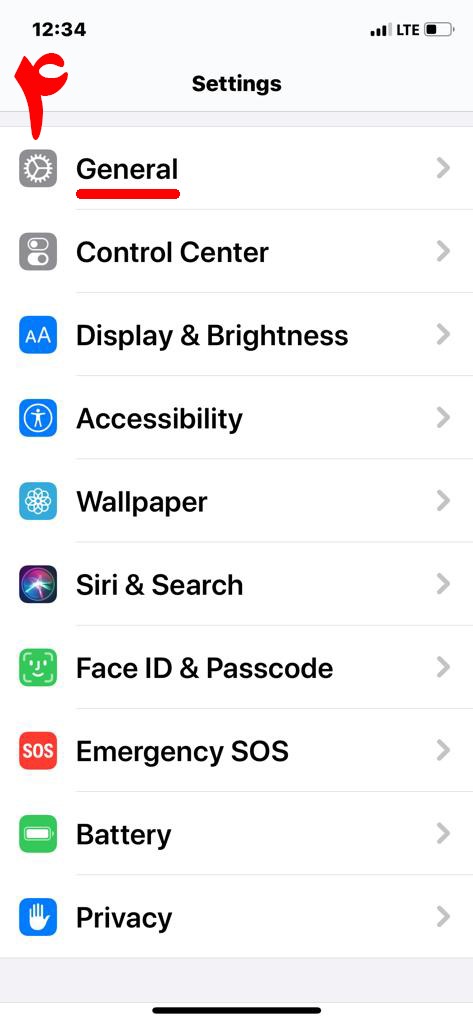In this image against a white background, there is a screenshot of a cell phone displaying the settings menu. At the top left, black text indicates the time as "1234." On the upper right, the status bar shows three out of four signal bars, the battery icon, and the "LTE" indicator.

At the center of the screen, the title "Settings" is displayed prominently in black text. Directly below the title sits a thin, gray horizontal line, demarcating the heading from the options below.

The settings options are listed as follows from top to bottom:

1. **General** - This option is underlined in red.
2. **Control Center** - Accompanied by a gray square on the left with two toggle icons inside.
3. **Display & Brightness** - Marked by a blue box with the letter "A" in white text.
4. **Accessibility**
5. **Wallpaper** - Featuring a light blue square on the left with a white snowflake-like design inside.
6. **Siri & Search**
7. **Face ID & Passcode** - Indicated by a green square with an illustrated face icon on the left.
8. **Emergency SOS** - Represented by a red square with white "SOS" text.
9. **Battery**
10. **Privacy**

The detailed layout and colored icons provide a clear and intuitive navigation interface for adjusting various settings on the cell phone.